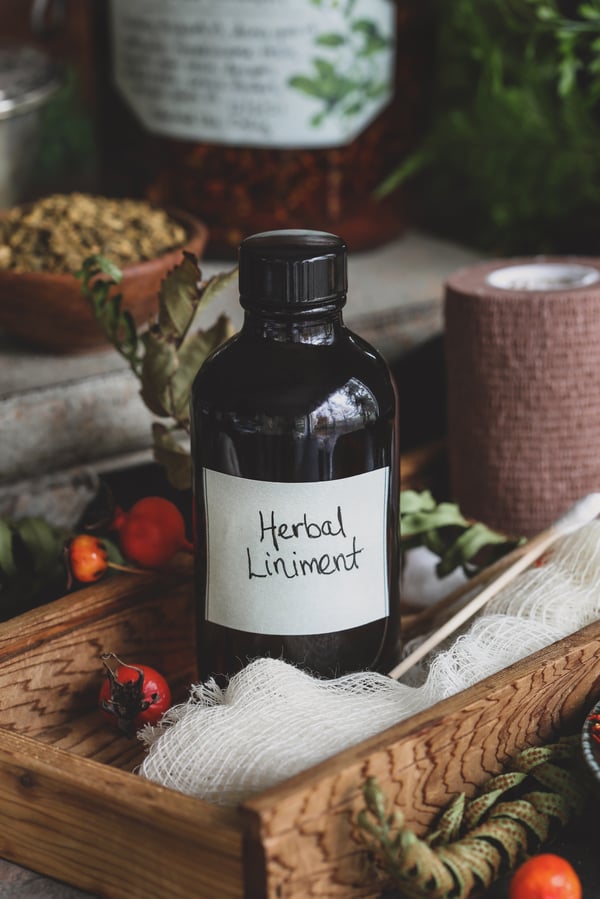This vertically rectangular, color photograph, likely taken indoors with natural light, primarily features a clearly staged setup. Central in the composition is a black glass bottle with a white, hand-drawn label reading "Herbal Liniment." The bottle, topped with a black plastic screw-on cap, sits in a small rectangular wooden box. Inside this box, alongside the bottle, are a couple of small red cherry tomatoes and some white gauze-like material, with an additional cherry tomato visible in the very lowest right-hand corner. To the upper left of the image, partially unfocused, is a wooden bowl filled with what appears to be a salad or possibly grains, accompanied by green branches. Also in the background, less clearly defined, is what seems to be a large glass jar containing red items, possibly pickled vegetables, and a roll of brown gauze. The setting of the photograph suggests careful arrangement likely intended to evoke a natural or rustic ambiance.